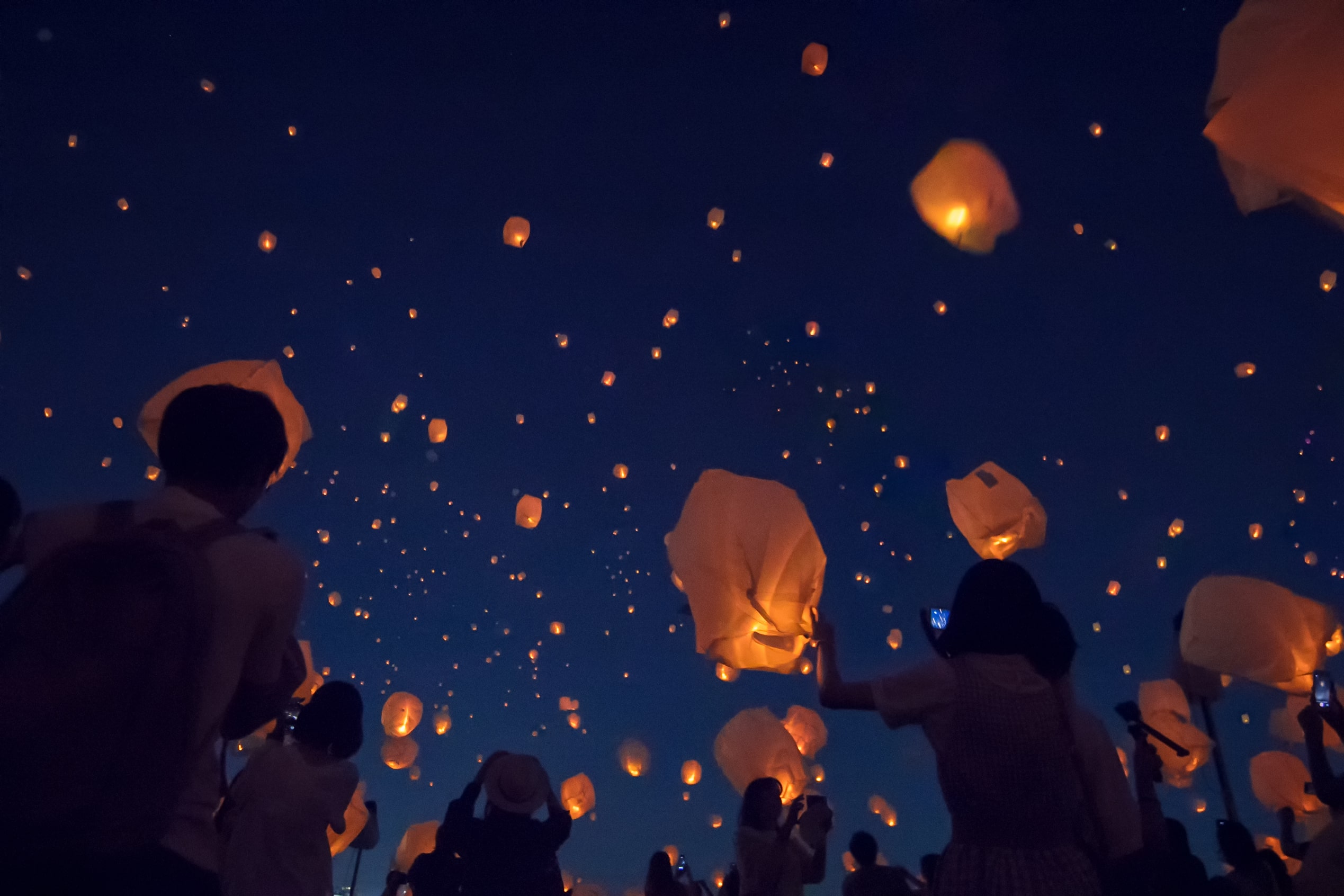In this captivating night scene, a large group of people is seen from behind, silhouetted against a dark blue and black sky. They are gathered to release lanterns with yellow glows at the bottom, creating a breathtaking spectacle. The photo, taken from the ground looking upwards, shows numerous lanterns already soaring high, dotting the sky with bright points of light. Some participants are holding selfie sticks and cameras, capturing the mesmerizing view, while others release more lanterns into the sky. The atmosphere suggests a communal event, possibly to commemorate a significant occasion, as the illuminated lanterns light up the lower portion of the sky, contrasting with the darker upper reaches. The scene is almost surreal, with the lanterns appearing like balloons, adding to the enchanting and solemn ambiance.